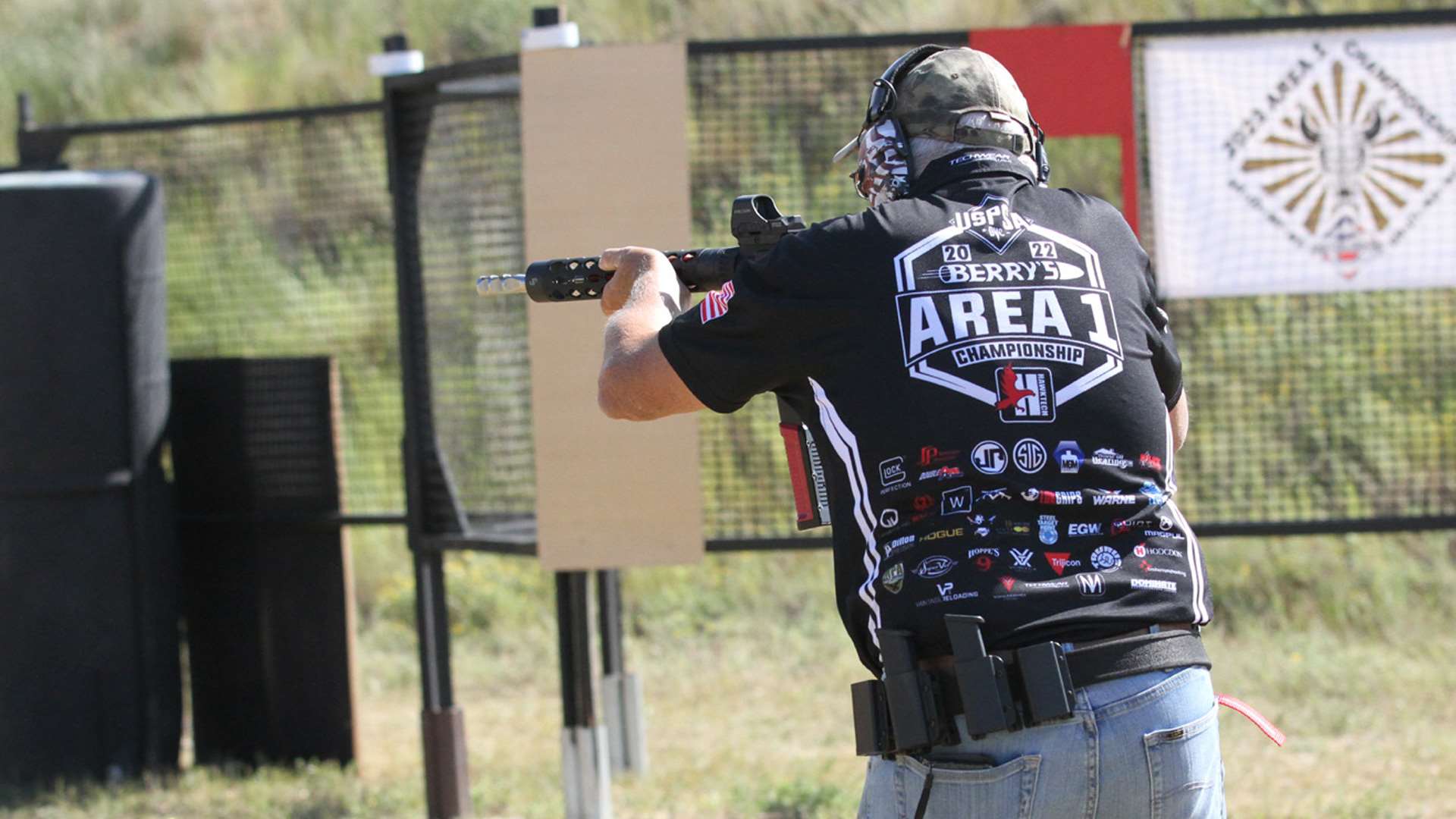In this vividly detailed image, a man is seen from behind at an outdoor shooting range, engaging in target practice with a massive firearm. He is sporting a black t-shirt emblazoned with multiple insignias including "Barry's Area 1 Championship" along with various sponsored logos on the lower back. On the right sleeve of his shirt, an American flag is prominently displayed. This marks the attire of the shooter, who is further outfitted with a camouflaged hat and protective earmuffs. His attire also includes blue jeans and a utility belt loaded with ammunition. The gun he is wielding is substantial, resembling a high-powered automatic rifle with a rotating barrel, suggesting significant firepower. Positioned beside him is a large black fence adorned with signs, one of which partially reads "2022 Area 1 Championship." The setting is bathed in natural daylight, revealing green grass beyond the fence and enhancing the clarity and vibrancy of the scene.